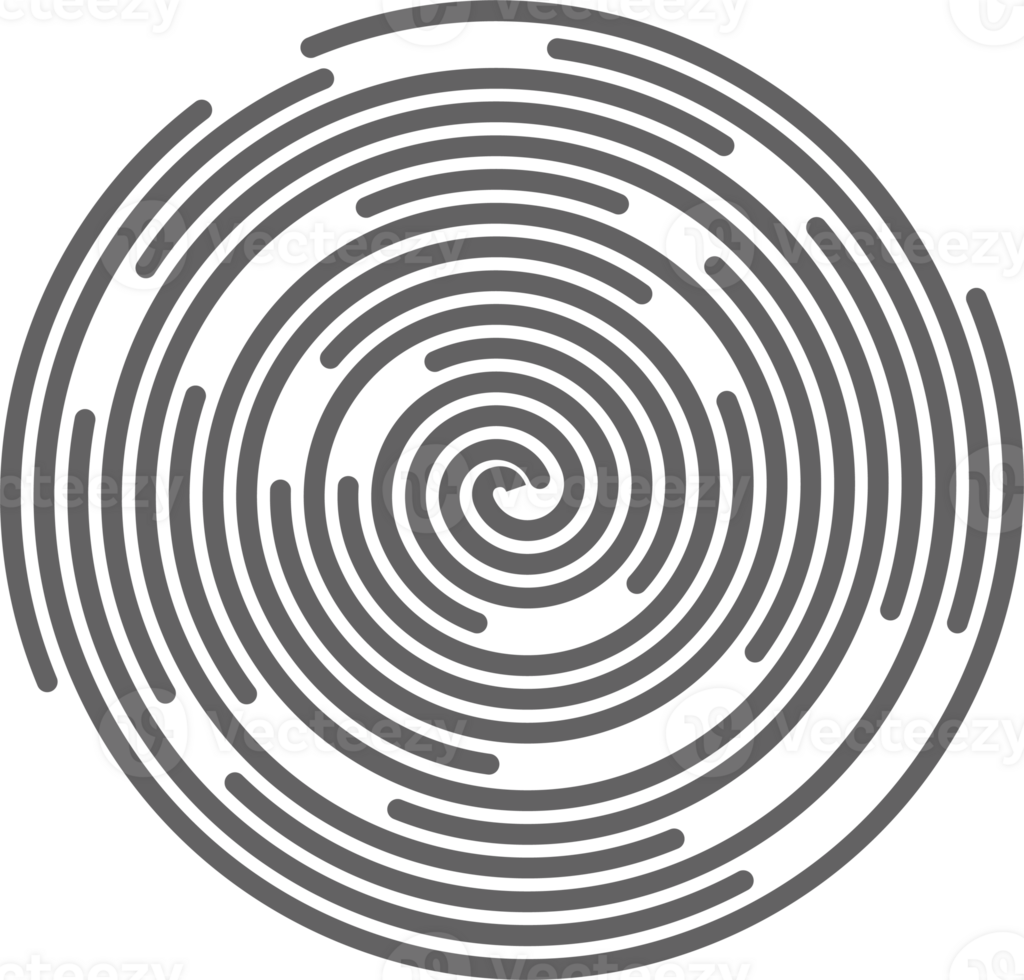The image showcases a detailed line drawing of a gray spiral with a circular pattern. The spiral design features alternating dark gray, almost black lines, and white spaces, creating an optical illusion reminiscent of imagery found in optical illusion books. The lines move in a clockwise direction from the outer edge towards a central point, giving a dizzying effect. The entire composition is overlaid with a barely legible watermark that reads "V-E-C-T-E-E-Z-Y," which appears translucent and covers the entire image. The background of the image is flat white, providing a stark contrast to the intricate spiral pattern. The design suggests a blend of different lengths of spaghetti, tightly wound into the spiral, with occasional breaks in between the lines, adding to its maze-like appearance.